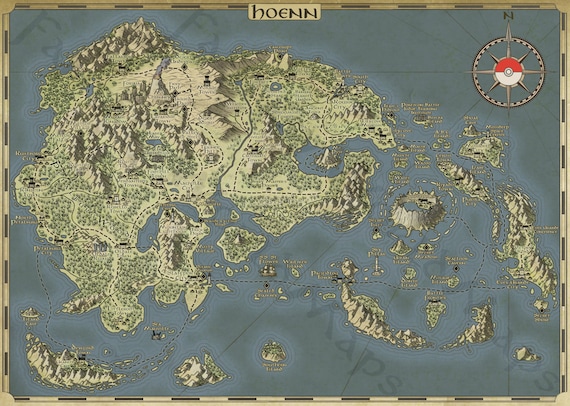This image depicts a hand-drawn, vintage-style map marked with the word "HOENN" at the top, rendered in an intriguing font that gives it an ancient, possibly even Celtic, appearance. In the top right corner, a large, red-and-white compass points north, featuring a symbol reminiscent of a Pokemon power icon. The map, partially visible and displayed on a dull, blueish-gray background, portrays a central mainland and surrounding islands, all detailed with various natural features such as mountains, trees, hills, and lakes. The terrain is richly illustrated with greenery, muted shades of green and beige for the land, and the water areas colored in different shades of muted blue and gray. Despite containing small labels, they are too blurry to read clearly and may be in a foreign language or archaic script. The map gives off an antiquated feel, suggesting it might represent a historical or fictional world from the distant past.